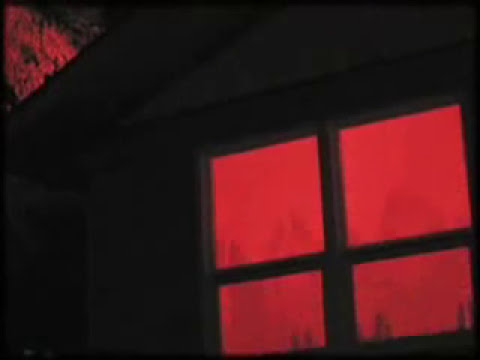This image is a detailed drawing depicting a dark, eerie interior of a room, creating an unsettling, almost horror movie-like atmosphere. The central focus of the drawing is a red-lit window with four panes, positioned in the bottom right corner of the rectangular image, starkly standing out against the otherwise black and dark gray background. The room appears shrouded in darkness, with minimal visible details due to the nighttime setting. Some barely distinguishable black shapes, possibly representing buildings or shadows, can be seen through the window, adding to the room’s creepy vibe. In the upper left corner, there is a mysterious red and black object, adding another layer of intrigue to the image. The room’s walls are not clearly visible, further enveloping the scene in an aura of mystery and vague unease.